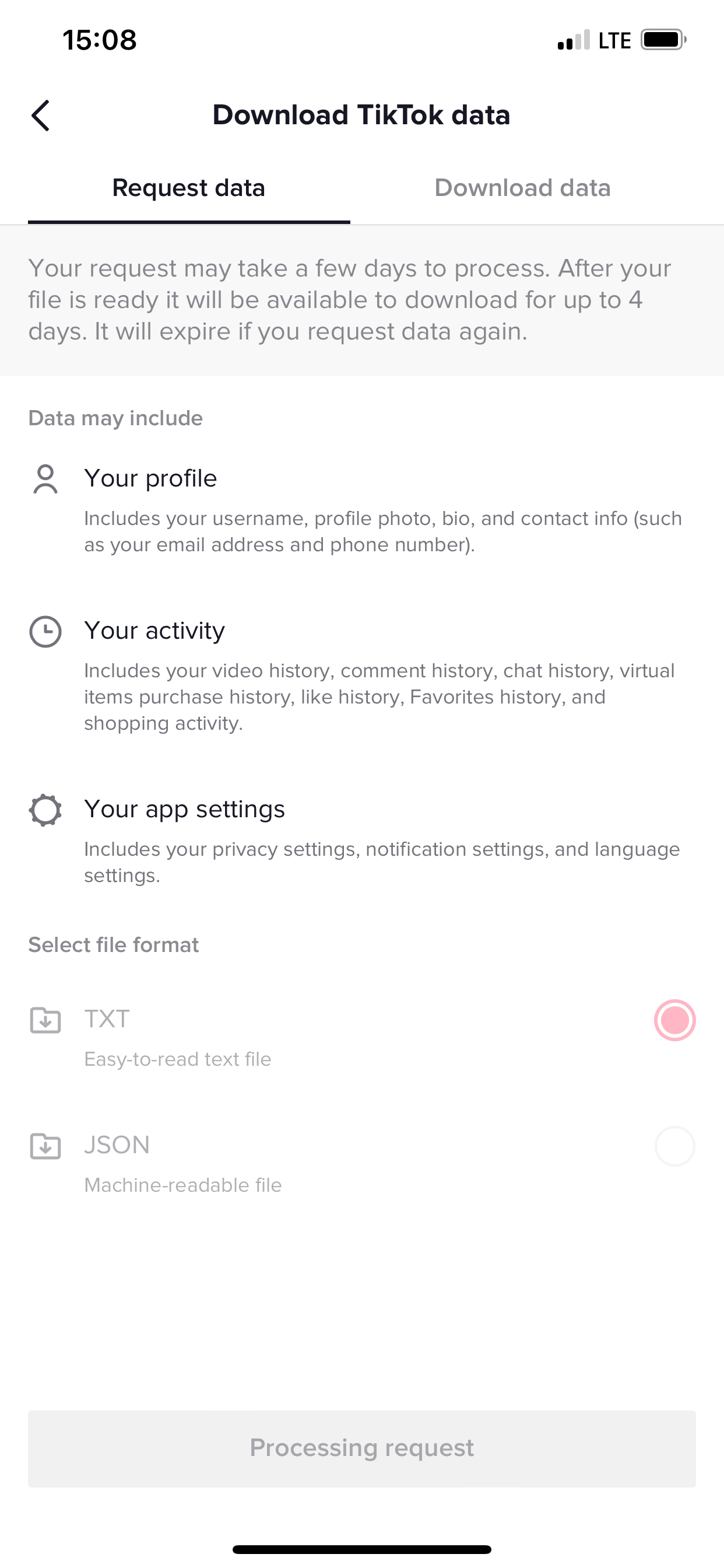This image is a cell phone screenshot showcasing the "Download TikTok Data" page. At the top of the screen, typical cell phone status icons are visible on both the upper left and upper right. Centrally aligned below them is the page title, "Download TikTok Data." 

There are two tabs situated under the title: "Request Data" and "Download Data." The "Request Data" tab is selected. Following this, a notice indicates, "Your request may take a few days to process. After your file is ready, it will be available to download for up to four days. It will expire if you request data again."

Under this note, there is a "Data may include" section divided into three paragraphs:

1. "Your Profile" – a concise description of the data related to the user's profile.
2. "Your Activity" – details about the data capturing the user's activities on the platform.
3. "Your App Settings" – a brief single sentence explaining the settings data.

At the bottom, there is a "Select File Format" section, indicating options for the user to choose the preferred format for their downloadable data file.